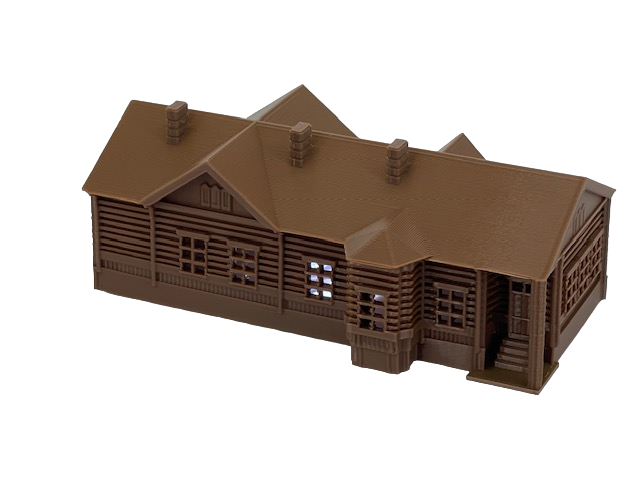This image, set against a seamless white backdrop that blends perfectly with the page edges, features a long, horizontally oriented log cabin house. The cabin’s exterior is characterized by its brown wooden planks with wide black gaps between them, resembling shaved logs. Prominently displayed are five vertical rectangular windows, each divided into six small panes by wooden bars. Notably, the second window from the right is part of a projecting dormer, adding dimension to the façade. A gable section appears on the left side of the house, accentuating the brown roof, which is topped by three distinct chimneys. Despite the seamless white background, the detailed elements of the house — from the slightly slanted positioning to the intricate window designs — stand out vividly, suggesting a possible CGI creation or a meticulously staged photograph. Highlighting a mix of browns, whites, blacks, and subtle grays and blues, this structure evokes the charm of a log cabin, potentially hinting at a children's playhouse but rendered in striking, lifelike detail.